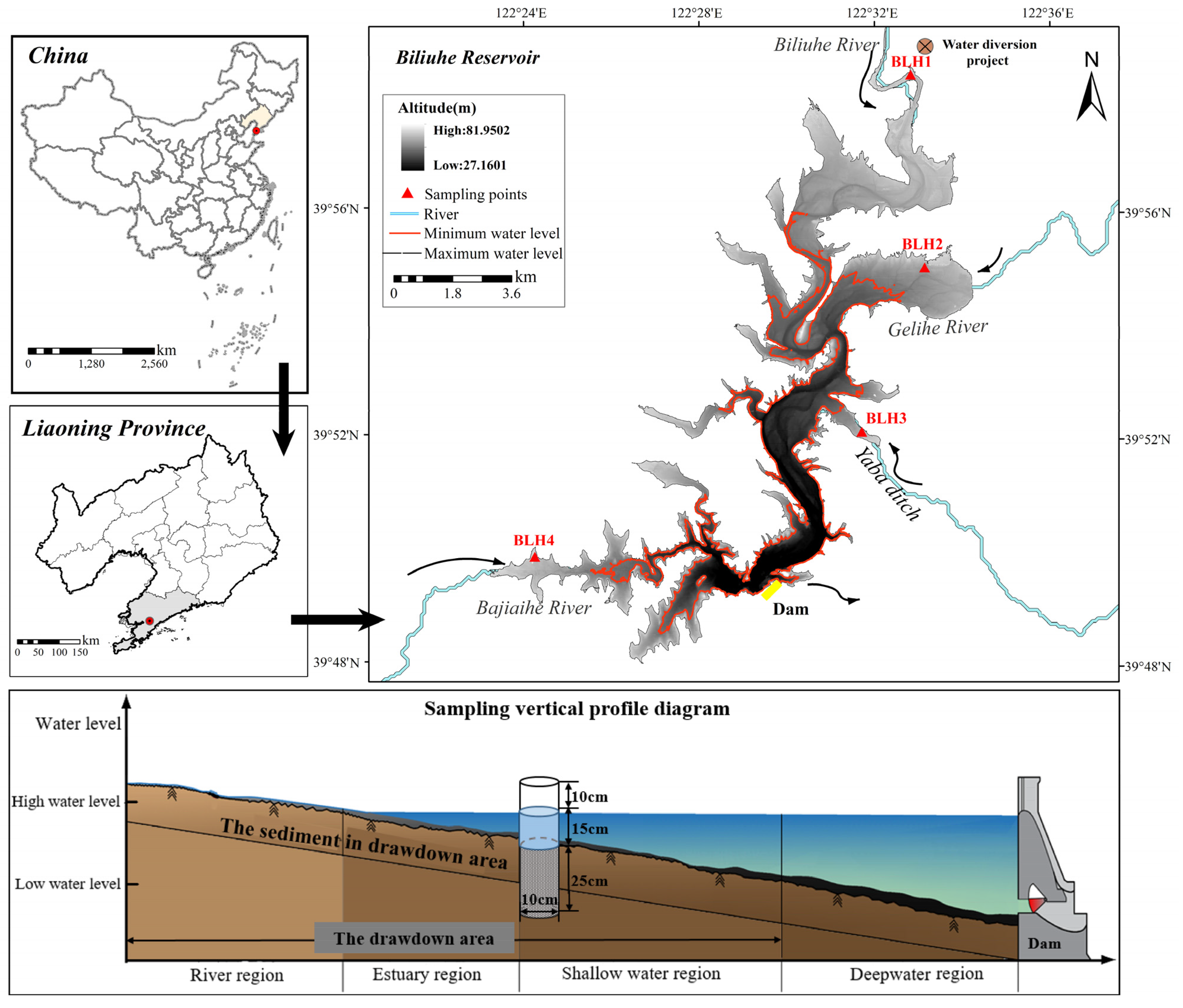This detailed illustration presents three distinct maps, each demarcated with black lines, showcasing geographical and hydrological data related to water flow in China. At the top left, a map of China features a red dot indicating a specific location. Below and connected by a downward arrow, the subsequent map details Lonin Province, also marked with a red dot at its bottom, showing further locational granularity. To the right, a third map labeled "Bulet Reservoir" details the water flow towards a dam, using brown to depict soil and blue for the water bodies.

Text annotations indicate sampling points as triangles, river regions in blue, minimum water levels in red, and maximum water levels in gray. The coordinate system includes specific latitude and longitude markings, enhancing spatial precision. A key is provided to clarify these symbols, and distance scales are noted in kilometers.

The diagram labeled "Sampling Vertical Profile" elaborates on the water levels and regions, showing a river region, estuary region, shallow water region, and deep water region. This section is enriched with a graph illustrating high and low water levels and detailed text indicating regions of different water depths and sediment data. Additional features include a black X marking the "Water Diversion Project" and several red and black arrows pointing towards various hydrological features such as the Baloo River and Yaba Ditch.

Overall, the illustration comprehensively visualizes how water flows from various sources to the Bulet Reservoir, facilitated by diverse keys and annotations for precise interpretation.